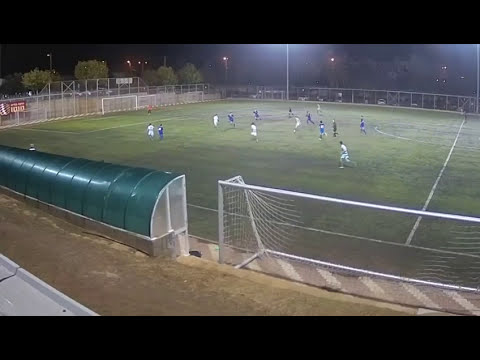The image is a small, rectangular, horizontal photograph that appears to be of a soccer field viewed from a distance, possibly from a live video or security footage exhibiting a slight fisheye lens distortion. The field is primarily green with white boundary lines and markings. In the foreground, there's a small dirt patch near the goals. Two teams are playing, one in white jerseys and the other in dark or black attire, but the players appear quite small due to the distance. The scene suggests a night-time game in a relatively small, empty stadium that looks like a school facility, encompassed by white fencing. The stadium has dark bands at the top and bottom of the image, and in the middle distance, it features a rounded roof structure which might be a dugout or team area. Behind the players, near the back, there are some bleachers which seem unoccupied. The setting includes a distant, possibly brown, track surrounding the field and some trees in the far background, signifying an outdoor environment.